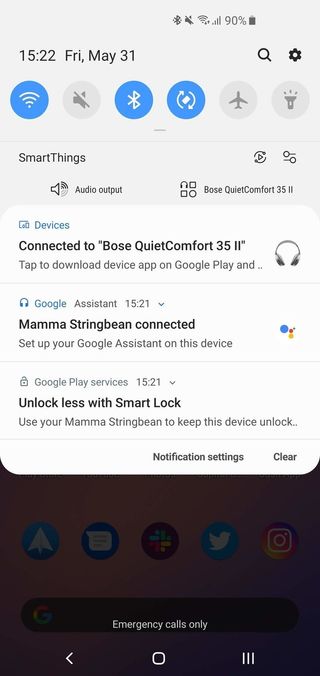In the image, a cell phone screen is depicted with various notifications and icons. At the top of the screen, the status bar shows the Wi-Fi icon, connection icon, and battery life at 90%. The current time is displayed as 15:22, along with the date, Friday, May 31st. Adjacent to the time are a search bar icon and a settings icon.

Below the status bar, there are six circular icons arranged in two rows. The first three icons from left to right include a Wi-Fi icon (lit up in blue), a mute icon (gray), and a Bluetooth connection icon (blue). The next three icons are a screen rotate icon (blue), an airplane mode icon (gray), and a flashlight icon (gray).

Below these icons, the screen reads "Smart Things" followed by "Audio output" and "Bose QuietComfort 35". Under this, it states "Devices connected to Bose QuietComfort 3511. Tap to download device app on Google Play" next to a headphones icon.

To the right, beneath this section, it mentions "Google Assistant, Mama Stringbean connected" with instructions to set up Google Assistant on the device. It also states, "Google Play Services 15:21, unlock less with Smart Lock. Use your Mama Stringbean to keep this device unlocked," followed by options for "Notification settings" and "Clear".

At the bottom of the screen, five app icons are displayed, with a note "Emergency calls only." Below this, there are the navigation icons: a back arrow, a square representing recent apps, and three vertical lines for accessing app switcher.

The image vividly presents a typical smartphone interface populated with various notifications, connectivity indicators, and navigation options.